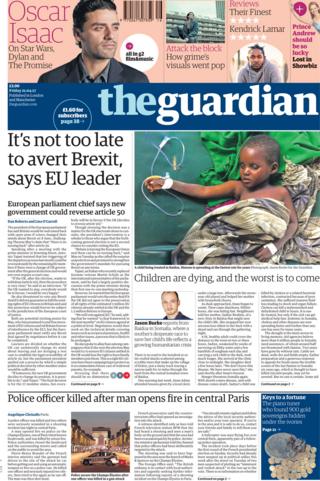The image is a news page brimming with a variety of headlines and photographs. In the top left corner, the bold text reads "Oscar Isaac on Star Wars, Dylan, and the Promise," accompanied by a headshot of the well-known actor Oscar Isaac and a barcode. Just to the right is a blurry photo of a person who appears to be standing in front of a fence, captioned, "Attack the Block: How Grimes Visuals Went Pop." Continuing to the right, the section labeled "Reviews" showcases several ratings, including "Their Finest" with four stars and "Kendrick Lamar" with five stars, adjacent to a picture of an African-American man wearing a hoodie.

In the top right corner, there is an image of a Caucasian woman with the headline, "Prince Andrew Should Be So Lucky, Lost in Showbiz." Spanning across the page is the prominent title, "The Guardian." Beneath this title, a headline reads, "It's not too late to avert Brexit, says EU leader. European Parliament chief says new government could reverse Article 50."

Dominating the right side of the page is a large, poignant photo of an African-American child connected to medical equipment, wrapped in a blanket with a medical bracelet on his left wrist. Below this image, the somber caption states, "Children are dying and the worst is to come." Underneath, another headline reports, "Police officer killed after man opens fire in central Paris," accompanied by an evocative photo depicting a scene from Paris.